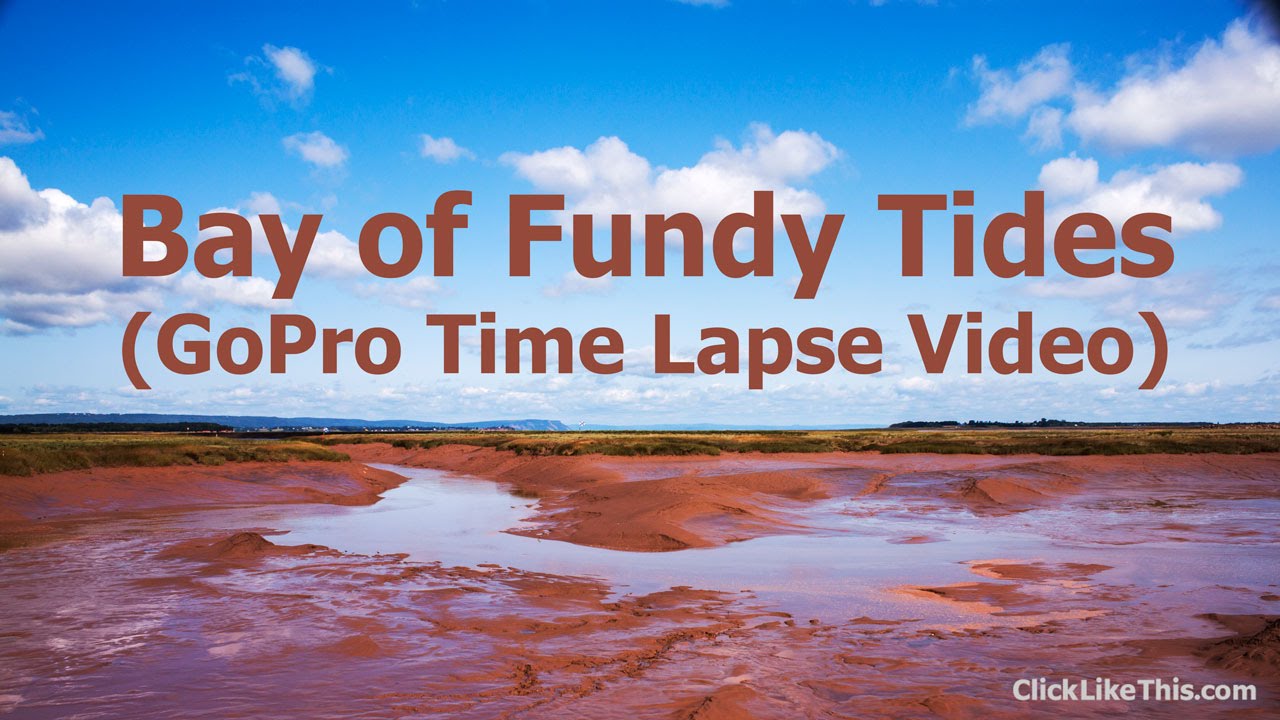The image is a digitally edited photograph showcasing a muddy landscape with shallow water patches, suggesting a low tide at the Bay of Fundy. It captures a wide vista with reddish-brown soil and some green vegetation on slightly elevated land. The background features a blue sky adorned with fluffy white clouds. Overlaying the upper part of the image is bold, brown text reading "Bay of Fundy Tides," followed by a smaller, similarly styled font within parentheses that says "GoPro Time-lapse Video." In the bottom right corner, white text displays "ClickLikeThis.com." The photograph, styled to resemble a GoPro time-lapse video, highlights the striking effects of the Bay of Fundy's tides.